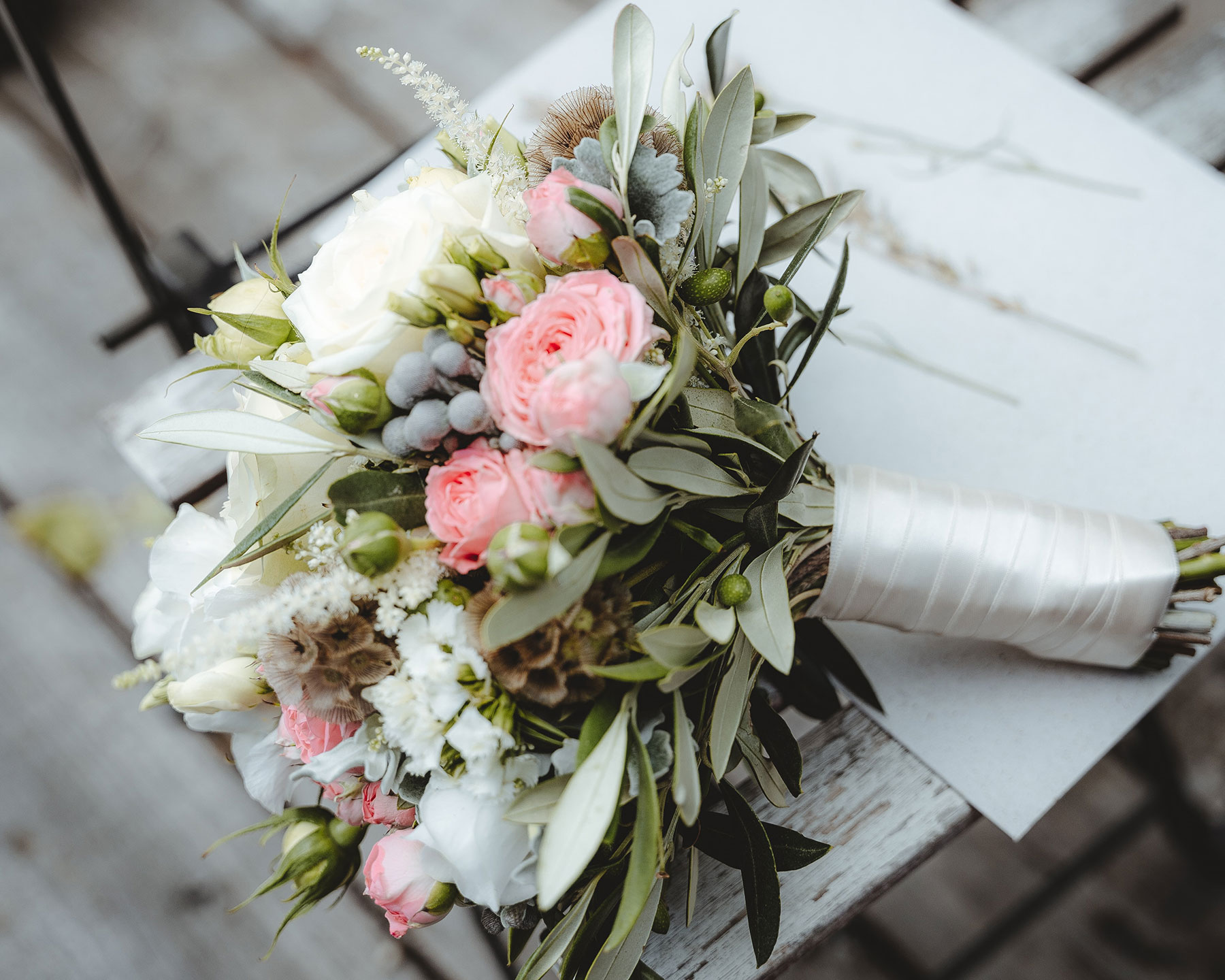In this photograph, an almost perfectly square image in landscape layout, we see a picturesque and elaborate bouquet of flowers resting on a rustic, whitewashed wood surface. The background, although intentionally blurred, reveals whitewashed wood textures that provide a charming, rustic ambiance. The bouquet is horizontally positioned with the stems wrapped in a shiny, white satin ribbon forming a handle on the right side, while the flowers bloom vibrantly on the left. The bouquet boasts an array of pink roses, cream-colored and white roses, pale green leaves, light blue berries, and baby's breath, creating a stunning and colorful display. Nestled beneath the bouquet is a white piece of paper, perhaps for wedding planning or a special occasion. This entire setup rests atop a wooden surface, possibly part of a simple patio chair with delicate, wrought iron detailing, suggesting an intimate, outdoor setting perfect for capturing the beauty of this exquisite floral arrangement.